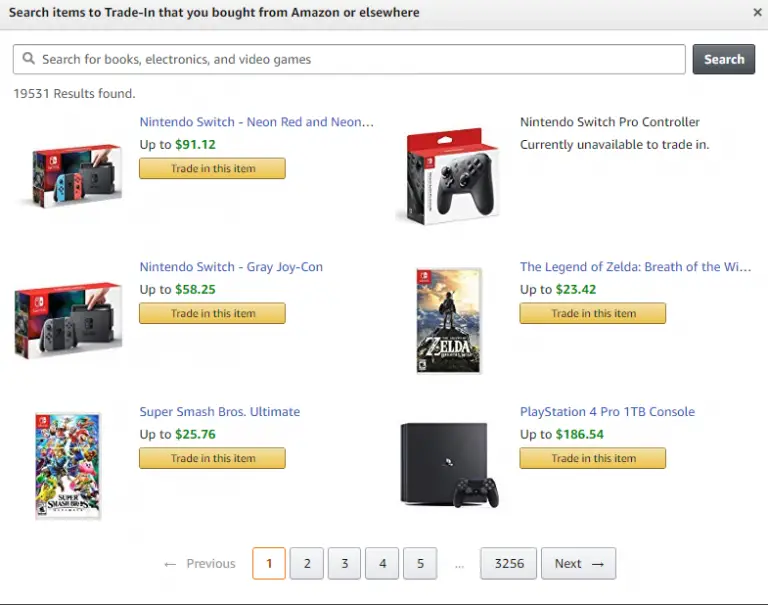The webpage features a detailed interface designed for trading in items. At the top, there is a prominent gray rectangle with bold black text that reads, "Search item to trade in that you bought from Amazon or elsewhere." Directly beneath is a search bar labeled "Search for books, electronics, and video games," accompanied by a black search button on its right.

On the left side of the page, there is a listing of items available for trade-in. The first item is a Nintendo Switch with blue and red Joy-Con controllers, accompanied by a beige-yellow "Trade in this item" button. Below that, a black Nintendo Switch is listed, also with a "Trade in this item" button. The third item in this column is "Super Smash Bros. Ultimate," which similarly features a "Trade in this item" button.

The right side of the page presents another list of items:
1. A Nintendo Switch Pro Controller in a box with a white base and a red top.
2. "The Legend of Zelda: Breath of the Wild" (though the title is partially obscured and reads "Breath of the Wi...").
3. A PlayStation 4 Pro, accompanied by an image of the console.

At the bottom of the webpage, navigation options are provided with "Previous" and "Next" buttons, enabling users to browse through different pages of trade-in items.